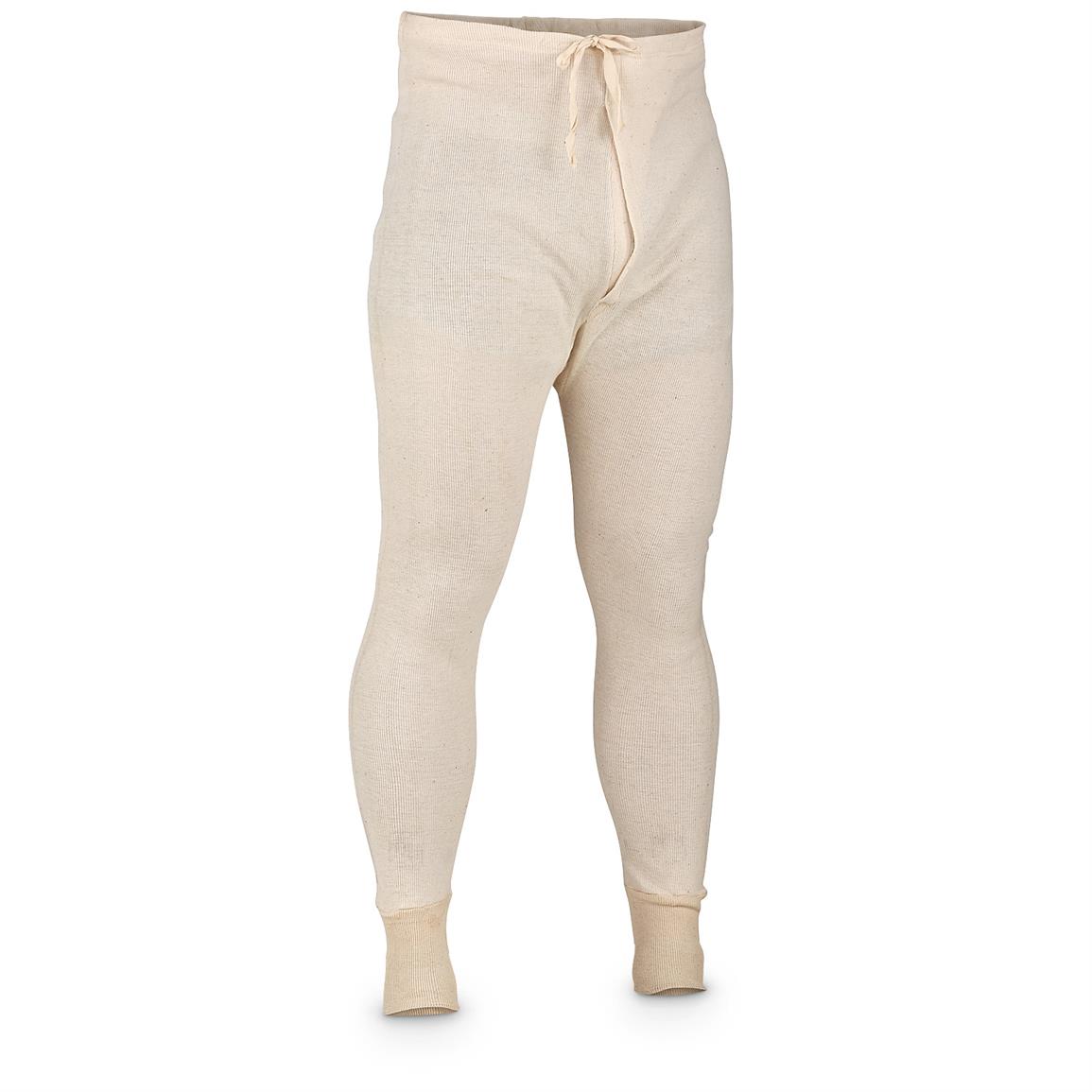The image is a high-resolution, color photograph featuring a pair of Long John pants, filling the entire frame against a seamless white background. Presented in portrait orientation, the pants are freeform, suggesting human contours without the presence of a model or mannequin. The Long Johns are a light cream color with the fabric showcasing a woven texture. They are designed with an elastic waistband tied in a bow for adjustable fit and include an opening near the crotch, indicating they are intended for male wear. The garment extends to the ankles, ending in slightly darker tan woven cuffs. This well-centered product photograph exemplifies realism and is likely intended for use in commercial settings such as websites or magazines.